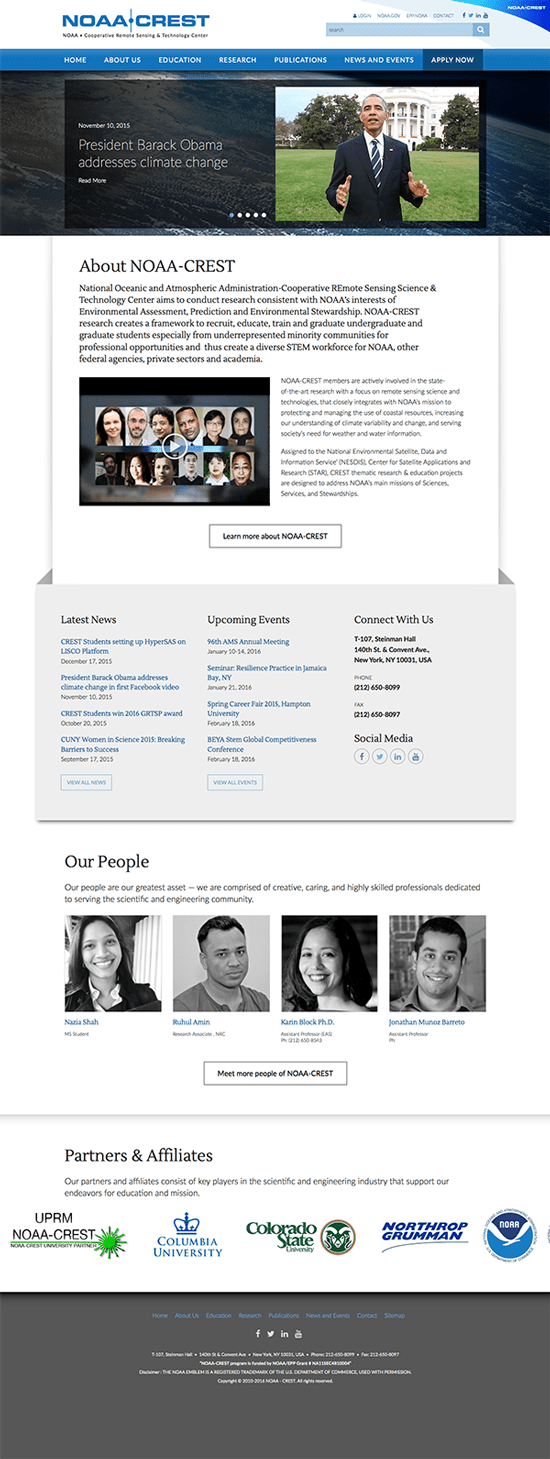In the image, President Barack Obama, dressed in a formal suit and tie, addresses the pressing issue of climate change from a podium outside the White House, which serves as the backdrop. The scene is part of a NOAA (National Oceanic and Atmospheric Administration) publication displayed on a website.

The website header features "NOAA" in blue with a vertical line separating "NOAA" from "CREST." The header includes options such as "Login," "Contact," and "Search." Below the header, a blue navigation bar offers links to sections like "Home," "About Us," "Education," "Research," "Publications," "News," "Events," and "Apply Now."

Beneath the navigation bar is a highlighted date, November 10th, 2015, signifying the day President Obama delivered his address on climate change. There's also a button labeled "Read More" for additional information about his speech and initiatives related to climate change.

Further down, the page describes NOAA CREST, the Cooperative Remote Sensing Science and Technology Center, which conducts research aligning with NOAA's environmental assessment, prediction, and stewardship interests. An embedded video explains NOAA's state-of-the-art research focused on remote sensing science technologies, supplemented by a "Learn More" button.

The webpage also features the latest news with four clickable links and lists upcoming events. Finally, there's a section to connect with NOAA CREST through phone or fax, a provided physical address, and profiles of key staff members: Nausea Shah, Ruchal Aman, Karen Block, and Jonathan Rito. Partner affiliates include Columbia University, Colorado State University, Northrop Grumman, and UPR MNOA CREST.